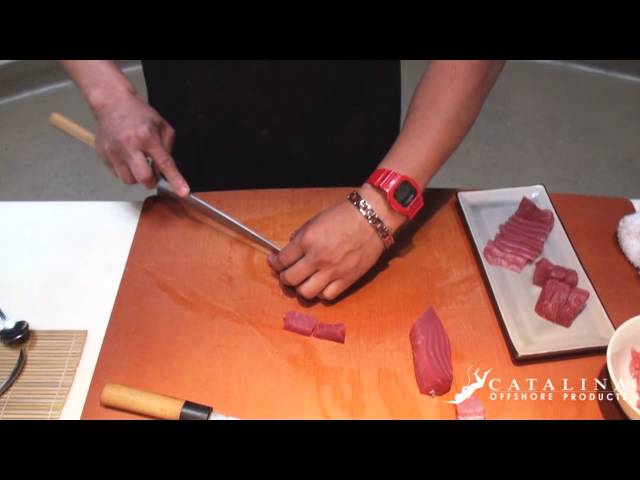In this image, a person, likely a chef, is meticulously slicing red meat on a large wooden cutting board. The person's left wrist is adorned with a red wristwatch and a bracelet. The chef is dressed in a black shirt, and his hands are the main focus of the image. He is wielding a long, sharp knife to cut the meat into smaller pieces. The cutting board dominates the middle of the frame, with a white rectangular plate already holding portions of the sliced meat to the right. To the left, there's a glimpse of a white countertop. The meat being prepared appears to be tuna, possibly for sushi. The bottom right corner of the image features a watermark: "Catalina Offshore Products," written in white text along with a symbol of a diver, signifying a professional seafood supplier. The overall image has a slight out-of-focus quality and includes black borders at the top and bottom. In the background, the gray floor is partially visible.